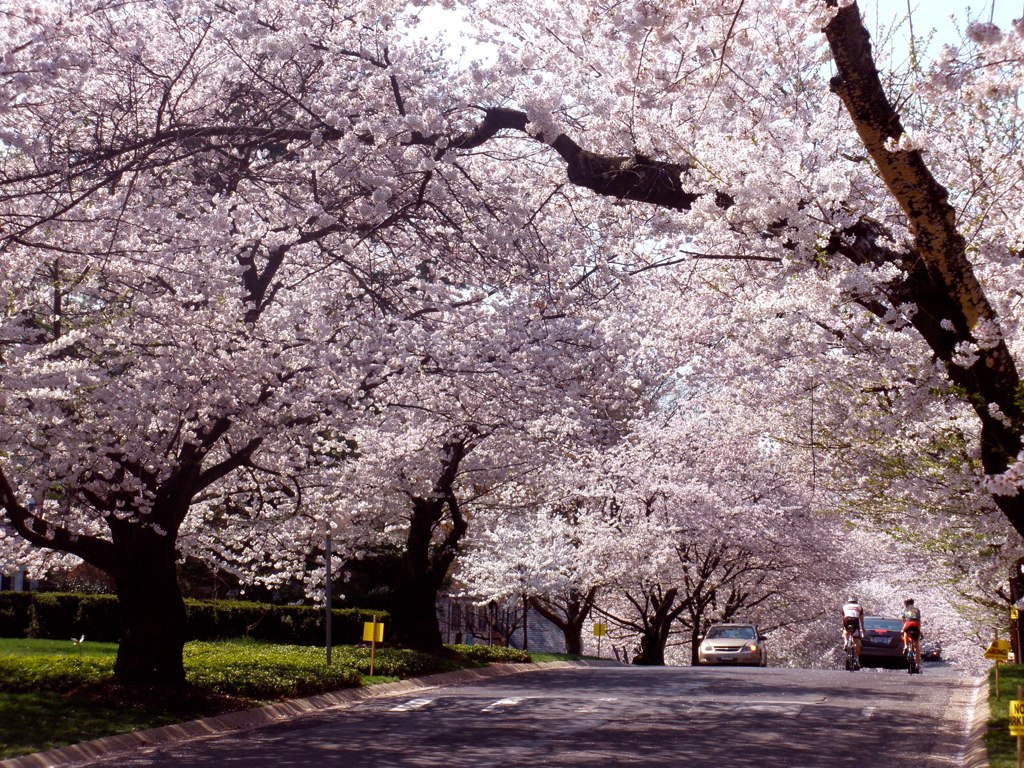The image captures a picturesque suburban neighborhood in full springtime bloom. The scene is dominated by a stunning, almost overwhelming display of blossoming cherry trees, their branches laden with thousands of delicate pink and white flowers, creating a canopy over the road. These flowers cover approximately 80% of the photo's upper portion. The trunks of these trees are dark brown, nearly black, and the sheer volume of blossoms gives the impression of a floral blizzard.

The road itself, a two-lane street, gently slopes upward and is bordered by grassy patches on both sides. Yellow "No Parking" signs are visible on these grassy areas. There are no sidewalks, just grass leading up to a sloped curb. On the road, a silver car approaches from the left side of the image, while on the right, another car is moving away, accompanied by two cyclists riding side-by-side. A glimpse of blue sky peeks through the upper right corner, adding a touch of brightness to the enveloping canopy of blossoms. Together, these elements create a serene and vivid springtime snapshot of a quiet neighborhood street.